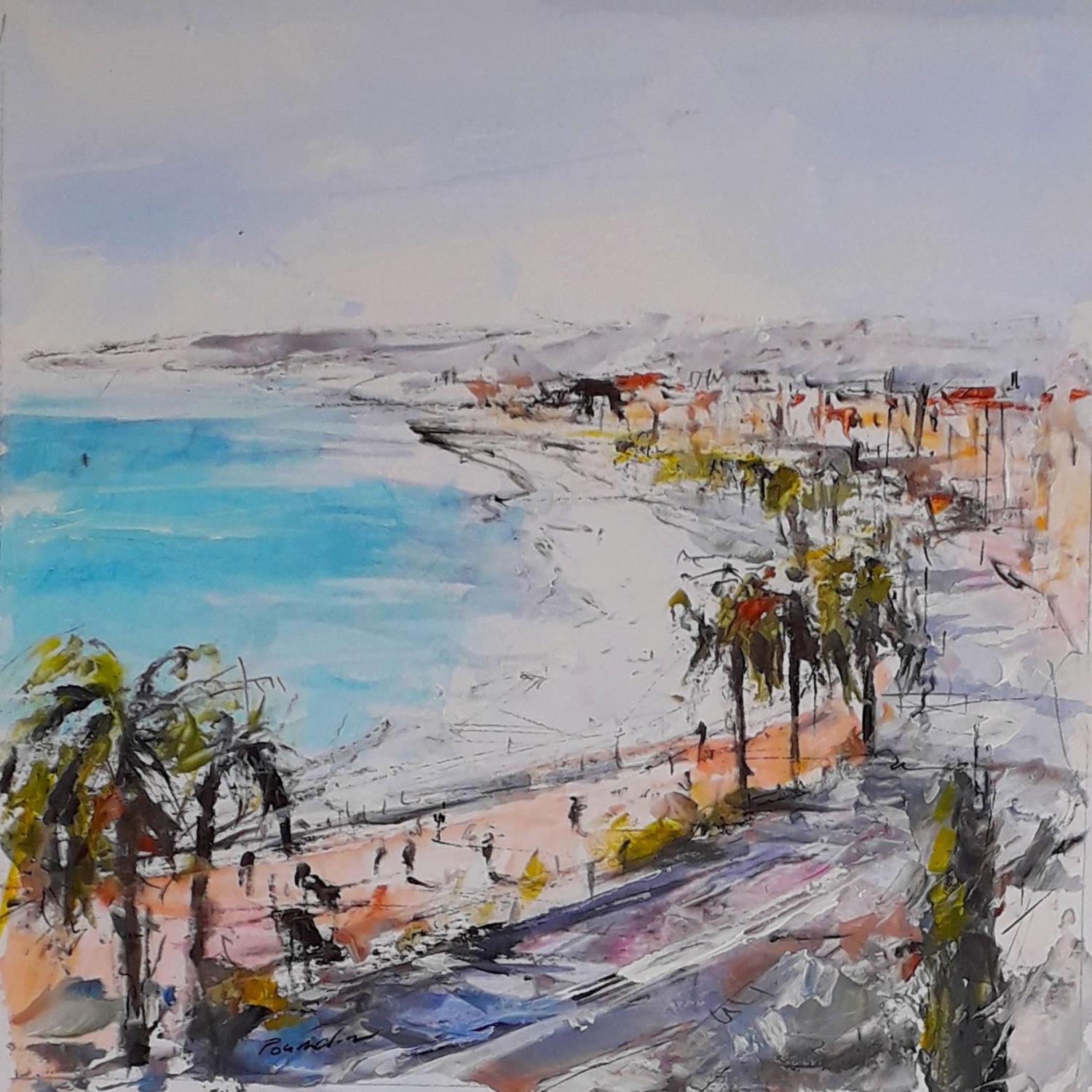This large impressionistic square painting, rendered without a border, captures a blurry yet vibrant coastal scene. The top portion, representing the sky, is primarily a soft blend of very light blues and predominantly white, suggesting clouds. Moving downward, the left-middle is dominated by a serene sea or large body of water painted in various shades of blue mixed with hints of white. Centered in the composition, there's a stretch of sandy shore depicted with a light brownish-gray hue. 

Scatterings of green and red leaves suggest tall palm trees emerging from brown trunks, notably curving around the lower left corner, and indicating lush vegetation along the beach. The right side teems with abstract representations of buildings painted with red, orange, and brown splotches, likely reflecting a small waterfront town. A series of mountains or hills form the distant background, their outlines hazy yet discernible under the mixed hues of gray and occasional blue sky above.

Despite the breadth of the scene, the depiction of people remains ambiguous with faint shadowy figures suggesting human presence on a brownish-orange road or boardwalk. A signature, though difficult to read, appears at the lower left, deciphered roughly as "P-O-U-M-A-L-I-Z."